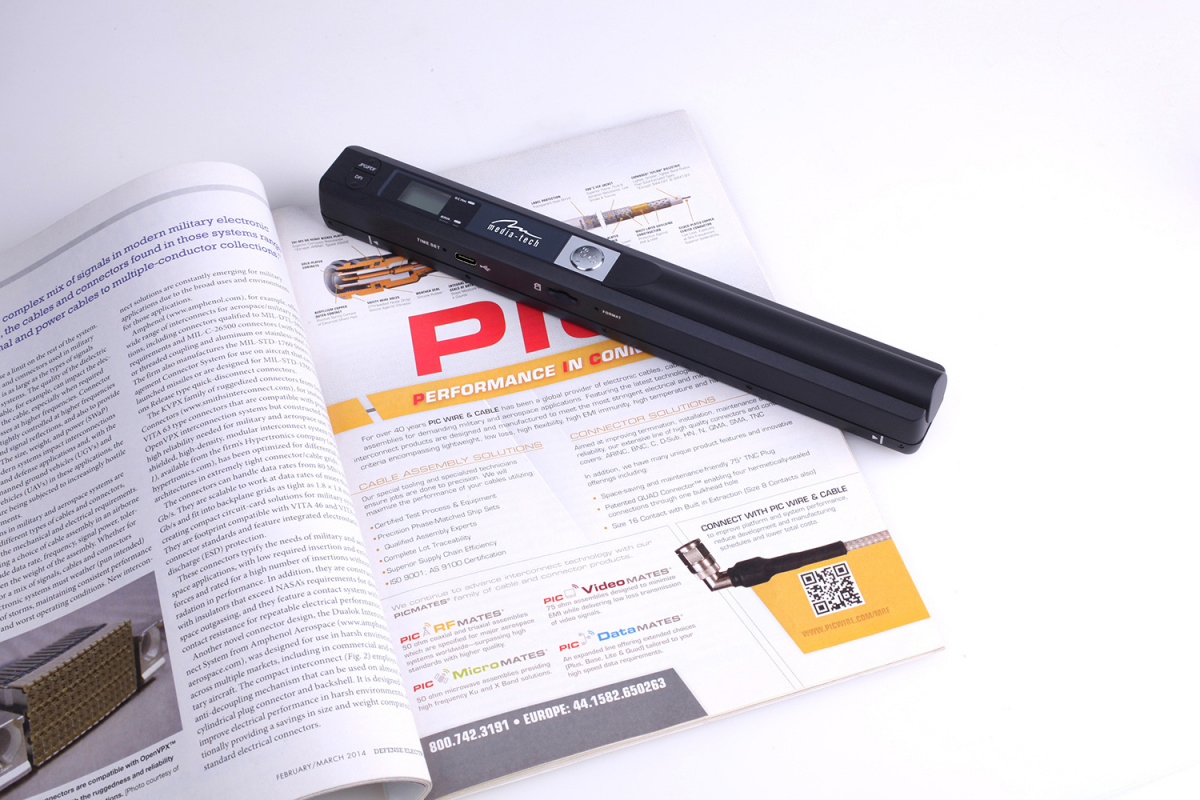The image displays an open magazine laid flat, revealing an advertisement page. The ad predominantly focuses on performance enhancements, featuring text like "performance" and "connect with PIC wire and cable," and displaying items such as PIC RF mates, PIC micro mates, PIC video mates, and PIC data mates. The ad also includes a QR code that directs to www.pickwire.com/MRI and lists contact numbers: 800-742-3192 and 44-1582-650-263 for Europe. The magazine showcases technical solutions with extensive text and diagrams.

Resting on top of the right-hand page of the magazine is a sleek, black device resembling a wand, about the width of the magazine page. The device features an LED screen, a couple of buttons, a memory card slot, and a USB port for charging, labeled as MediaTek. This gadget appears to be a portable scanner, designed likely for scanning magazine pages effortlessly by gliding over them.